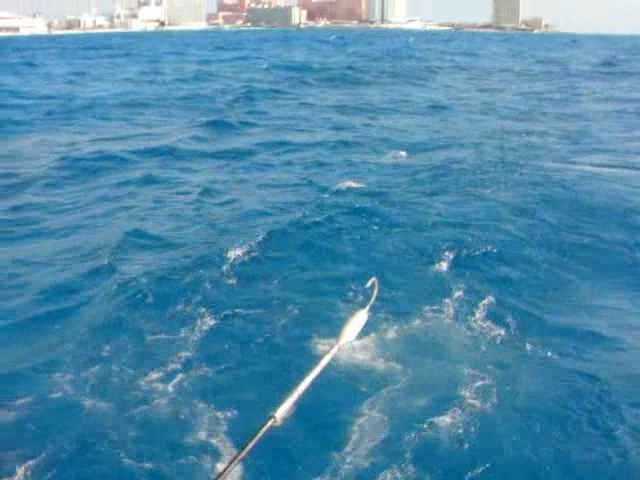This slightly faded, full-color photograph captures a scene aboard a boat at sea near a beach resort. The primary focus of the image is the expansive view of the dark blue ocean, which exhibits notable waves and white foam from the boat's wake, suggesting movement. In the bottom left corner of the photograph, a long metal hook attached to a rod extends outward, presumably used for deep-sea fishing. At the upper portion of the image, the distant shoreline features several indistinct tall buildings, possibly high-rises or large condos. The photo's composition gives a sense of the vastness of the ocean, emphasizing the predominance of water in the scene, with only a small segment dedicated to the distant shoreline and skyline. Additionally, there is a dark shape in the upper right corner that remains unidentified, hovering near the water’s surface.